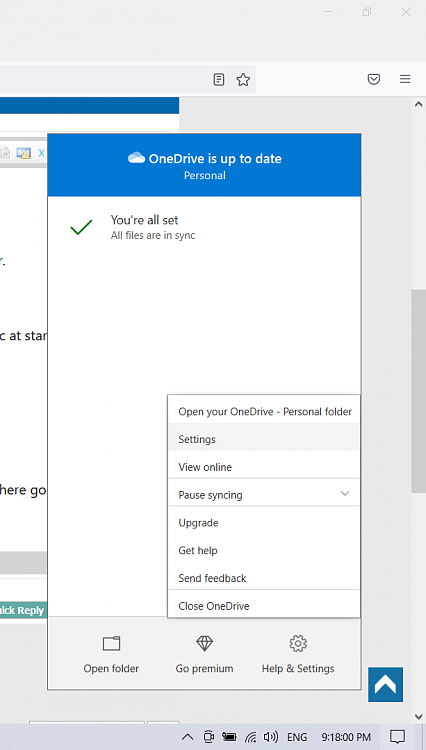The image depicts a OneDrive pop-up window against a greyish-white background, originating from a website. Dominating the center of the page, the pop-up features a distinctive blue bar, about an inch thick, running horizontally across its top. Centered within this bar is a cloud icon, adjacent to text stating, "OneDrive is up to date," followed by the word "Personal."

Below, on a white backdrop, a green check mark to the left is accompanied by the reassuring message, "You're all set." Further text confirms, "All files are in sync." Extending towards the bottom right-hand corner of the pop-up are various menu options listed vertically. These include: "Open your OneDrive-Personal folder," "Settings," "View online," "Pause syncing" (with a corresponding drop-down arrow), "Upgrade," "Get help," "Send feedback," and "Close OneDrive."

Underneath this menu, located on the left-hand side, are three icons with respective labels. The first, an icon resembling a folder, is labeled "Open folder." Adjacent to it is the image of a diamond, labeled "Go Premium." Lastly, an icon of a gear signifies "Help and settings."

The lower portion of the page, partially obscured by the pop-up, reveals a series of icons and information. At the center bottom is a black arrow pointing upwards, followed by an icon of a video camera, an unidentified black icon, an icon linked to ride-price strength, and a volume control icon. On the far right, the text "ENG" denotes language settings, alongside the time display reading "9:18 PM."